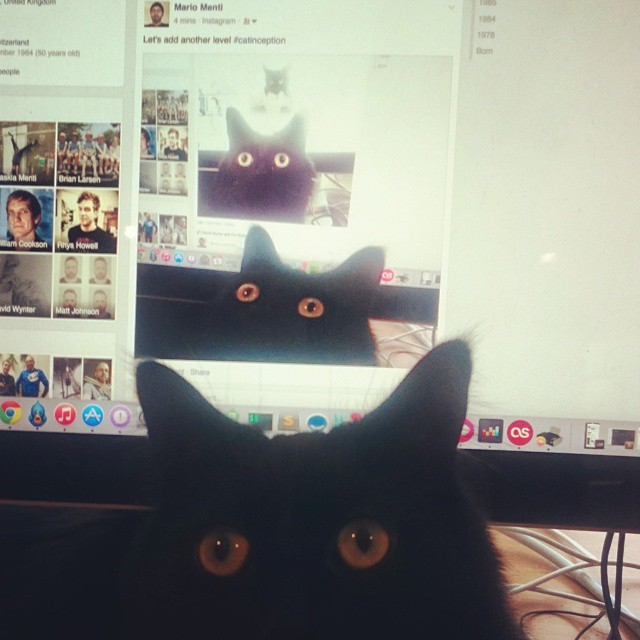The photograph captures a visually intriguing scene where a black cat with striking amber eyes is featured prominently in the lower portion of the image, primarily showcasing its head. The setting includes a computer monitor immediately behind the cat. The monitor displays an Instagram homepage, indicated by the visible username “Mario Mantel” and various icons. The image cleverly replicates the infinity mirror effect by showing the cat in front of the monitor, which repeatedly displays the same image of the cat in front of the monitor in a series of recursive frames, extending this visual sequence about four times. The dark, close-up nature of the photo emphasizes the cat’s eyes and adds depth to the recurring images, while cords connecting to the monitor are visible in the lower right. Additionally, the screen features several smaller profile images and icons on the left side, enhancing the detail and complexity of the composition.